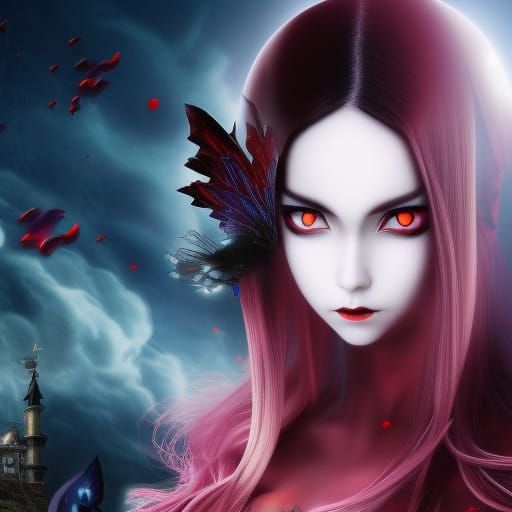This AI-generated image features a close-up of a mysterious and somewhat sinister-looking woman with striking details. Her face is pale white, framed by long, straight hair that fades from reddish-purple to light purple at the tips. Her eyes are mesmerizing with cat-like orange and red pupils, accentuated by heavy eyeliner. She has pink lip gloss highlighting her small lips. A leaf-like object, purple in color, adorns the left side of her hair near her eye. Notably, her neck appears hidden, completely enveloped by her long flowing hair. In the background, a dark blue sky looms with ominous blood splatters and swirling dark clouds. There are also hints of flying creatures within the clouds. At the lower left corner of the image, a manor or house with a tower, brown in color, faintly stands under the surreal, eerie setting.